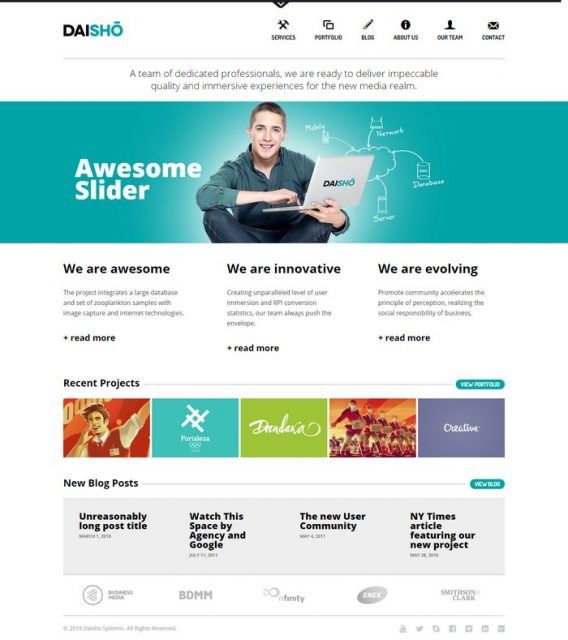Here is a detailed and clean descriptive caption for the image:

"The webpage features a white background with the company name 'DAI' in black letters and 'SHO' in blue letters. At the top of the page, there is a menu bar with the following visible options: Services, About Us, and Contact, with additional options too small to discern. Below the menu, a bold headline reads, 'A Team of Dedicated Professionals,' followed by a subheading that states, 'We are ready to deliver impeccable quality and immersive experiences for the new media realm.' Beneath this, a prominent blue box labeled 'Awesome Slider' showcases an image of a person working on a laptop.

Further down, the page highlights three core company values: 'We are Awesome,' 'We’re Innovating,' and 'We’re Evolving,' each accompanied by a 'Read More' link and a paragraph of descriptive text. The sections are followed by headers for 'Recent Projects' and 'New Blog Posts.' At the bottom corners of the page, various company logos can be found, alongside social media links, providing additional navigation and connection options."